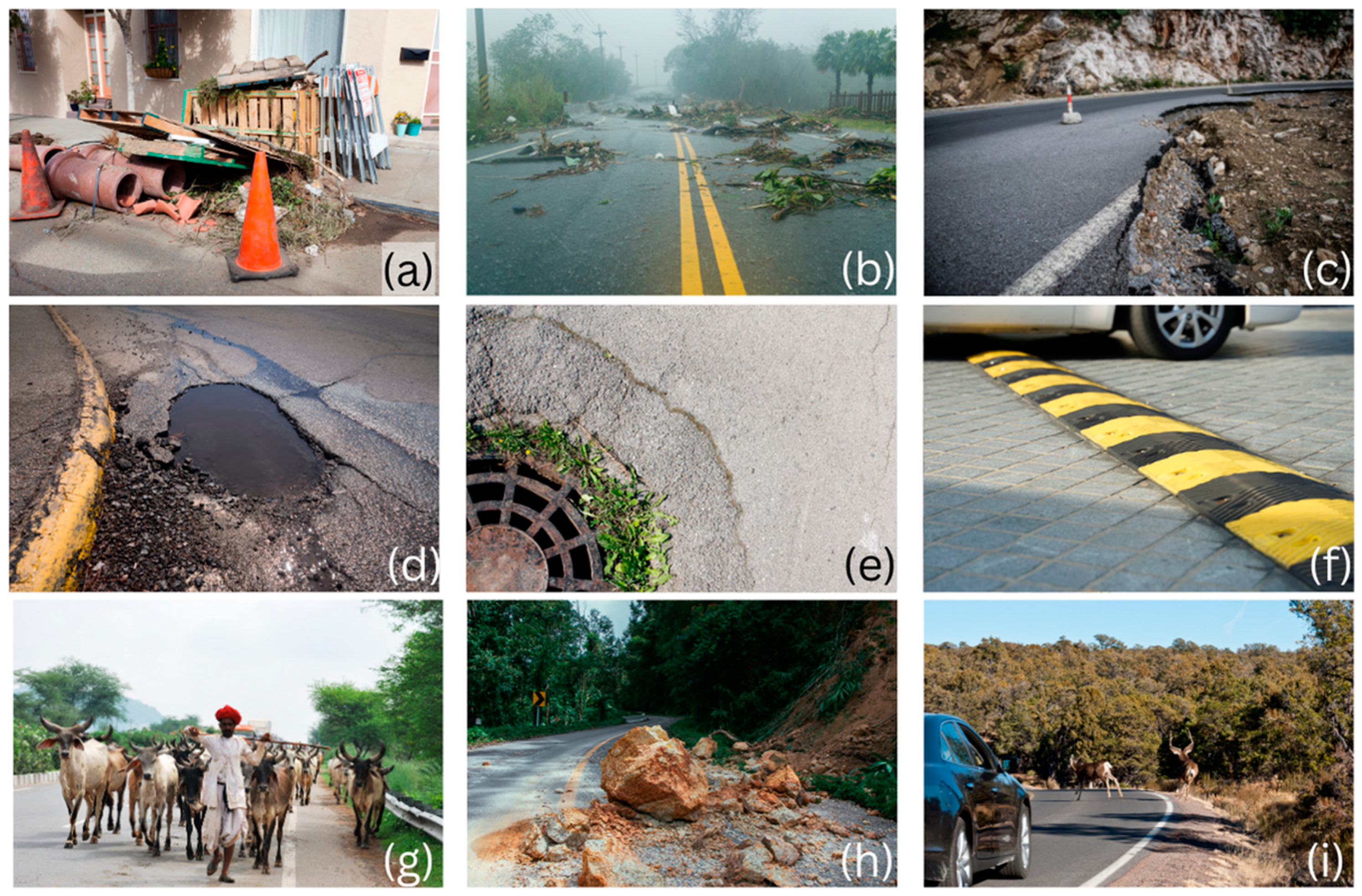The image is a composite made up of nine horizontally rectangular, full-color photographs, organized in a 3x3 grid layout without any borders but separated by distinct vertical and horizontal lines. Each photograph is labeled in the lower right-hand corner with a letter, A through I, in white text, except the top-left which is in black. The photographs depict a variety of road hazards and situations, each in vivid detail:

- **A**: Depicts a construction zone with various debris including wooden pallets and pipes laid on the ground, orange traffic cones surrounding the area, and a house visible in the background.
- **B**: Shows a two-lane road with a double yellow line, littered with fallen tree debris, indicating the aftermath of a storm.
- **C**: Features a curved mountain road where a section of the asphalt has eroded away, exposing the dirt underneath.
- **D**: Displays a large pothole located near a curb on the side of the road.
- **E**: Presents a drainage hole with visible cracks and grass growing around it.
- **F**: Illustrates a black and yellow speed bump situated on a gray, cobblestone-like road.
- **G**: Captures a man in white attire leading a herd of oxen, some yoked together, down a paved road.
- **H**: Shows a road obstructed by large boulders following a landslide.
- **I**: Features a few deer crossing a road in front of a car.

This detailed photographic collage emphasizes various types of road hazards, providing a realistic representation of each scenario.